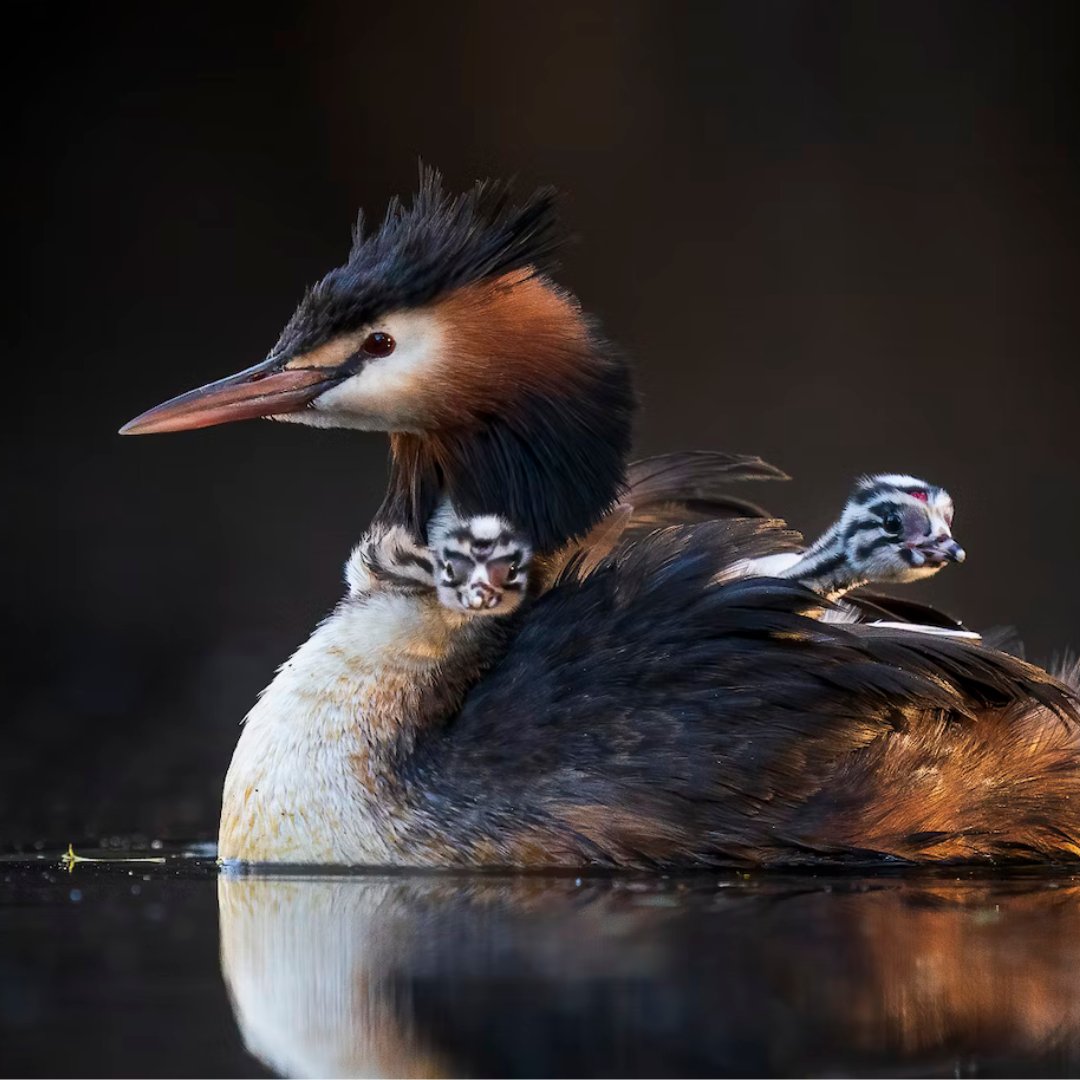The image displays a serene scene of a swan-like bird, likely a duck, gracefully swimming in calm, dark water that mirrors its form. The bird, central to the image, is characterized by its predominantly white body with black feather accents. Its head features a mix of black and white, with a striking red patch on its face and dark red to orange beak. Notably, it has red eyes and a fluffy black crown of feathers on its head. Two baby birds accompany the adult—one rides on its back, while the other seems nestled around its neck. These ducklings share the black and white color pattern of the adult. Sunlight from the right side of the image casts a golden reflection on parts of the bird's wing, adding warmth to the water's dark surface. The photograph is highly detailed, suggesting it was captured with professional equipment, effectively capturing the intimate and tranquil moment.